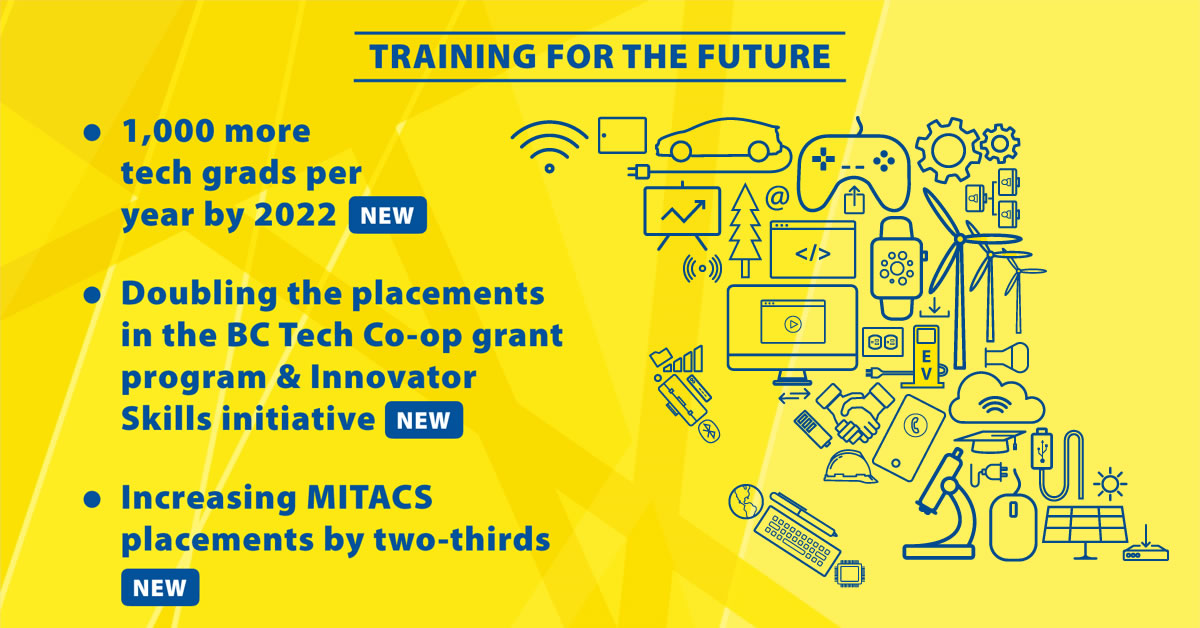The infographic titled "Training for the Future" is a rectangular, horizontally-oriented design featuring a predominantly yellow background with abstract, geometric shapes and various shades of yellow. Bold blue sans-serif text appears at the top, capitalized and framed with horizontal lines above and below, reading "TRAINING FOR THE FUTURE". 

On the left side of the image is a list with three blue bullet points, each accompanied by a rounded blue badge labeled "NEW". The bullet points read:
1. 1,000 more tech grads per year by 2022
2. Doubling the placements in the BC Tech Co-op Grant Program and Innovator Skills Initiative
3. Increasing MIT ACS placements by two-thirds

The right side of the graphic features a collection of blue line illustrations depicting various tech-related symbols, including a handshake, computer monitor, video game controllers, electric cars, Wi-Fi symbols, microscopes, mice, USB cables, graduation hats, windmills, smart watches, connected cogs, and networking icons. These illustrations contribute to the overall tech-focused theme of the infographic.